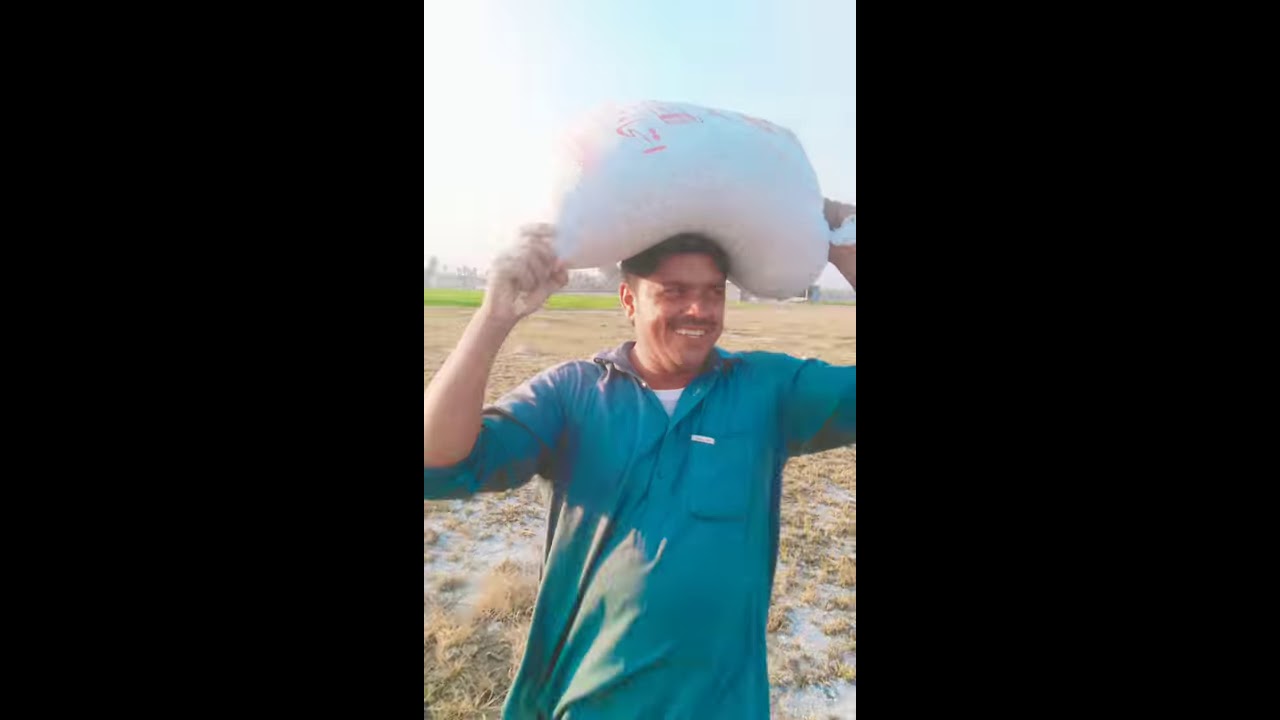The image captures a man with short black hair and a black mustache, wearing a blue shirt with a white undershirt beneath it. He is standing in a bright outdoor setting, holding a large white sack with pink writing, resting on top of his head. The man has a tan complexion and is smiling goofily off to the right. The background features a mix of dry sand and brush immediately behind him, transitioning into lush green grass further back. The sky above is bright with a hint of light blue down the middle. The photo appears to be taken with an older camera, evidenced by its lower quality and two large black vertical lines running down each side, suggesting it might have been cropped similarly to a smartphone video. There are no other people, animals, or readable text visible in the image.